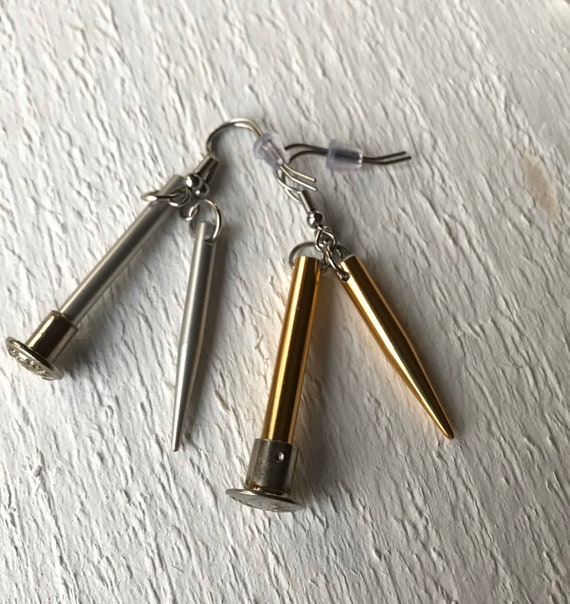The image shows four small metallic objects laid out on a white, textured surface that appears to be a painted table or soft material. These objects vary in color; two are gold, and two are silver. They are organized into pairs: each color features one object with a rounded head and another that tapers to a point. Each pair includes a stainless steel-like silver piece and a brass-like gold piece, all attached by rings of metal to metal hooks, possibly indicating they are meant to be hung or carried. These objects resemble a combination of defensive tools and artistic jewelry, like earrings, with each pair suspended by hooks and backing resembling traditional earring fastenings. Their exact purpose is unclear, but they suggest a mixture of functionality and ornamentation.